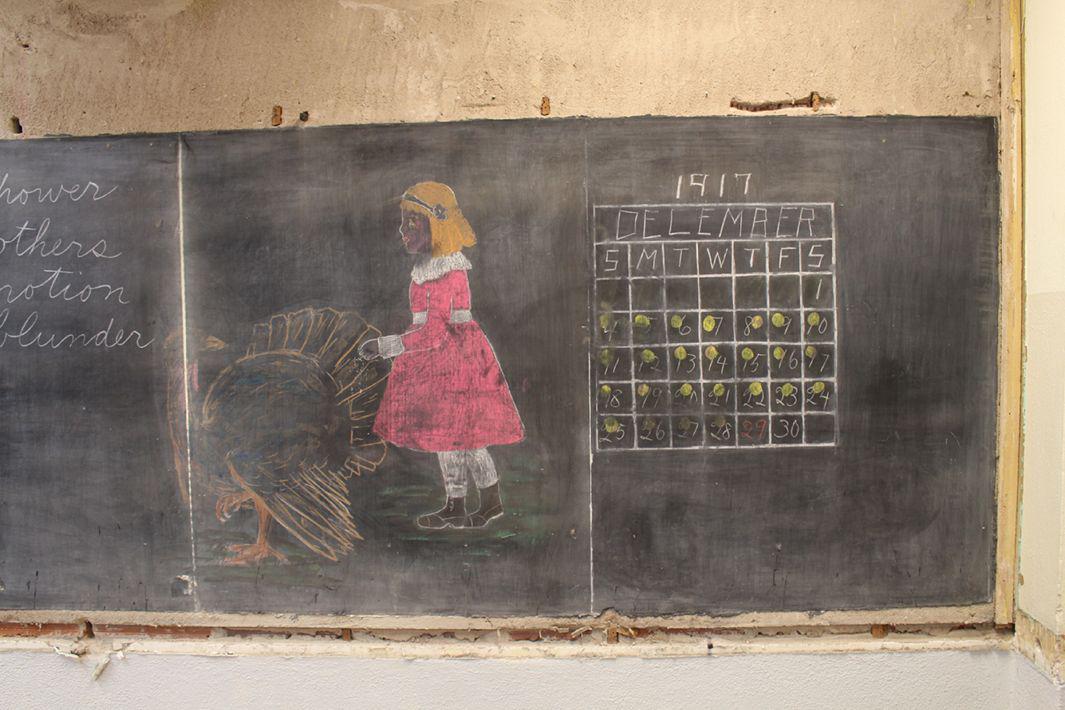The photograph features an old slate chalkboard mounted on a rough, tan-colored wall. The chalkboard is divided into three distinct sections. The left section has multiple cursively written words in chalk, with "shower," "notion," and "plunder" being partially visible. The middle section contains a detailed sketch of a turkey alongside a young girl. The turkey is primarily drawn in white chalk with orange legs, and the girl wears a pink dress with a white collar and belt, black shoes, white stockings, and has dark skin and yellow hair adorned with a black band. The rightmost section features a square-shaped calendar dated December 1917, with the days of the week labeled "S-M-T-W-T-F-S." Each date is marked by a small yellow circle, potentially indicating weather or events. The entire scene is set against a backdrop that captures the dusty essence of a vintage classroom or teaching space.